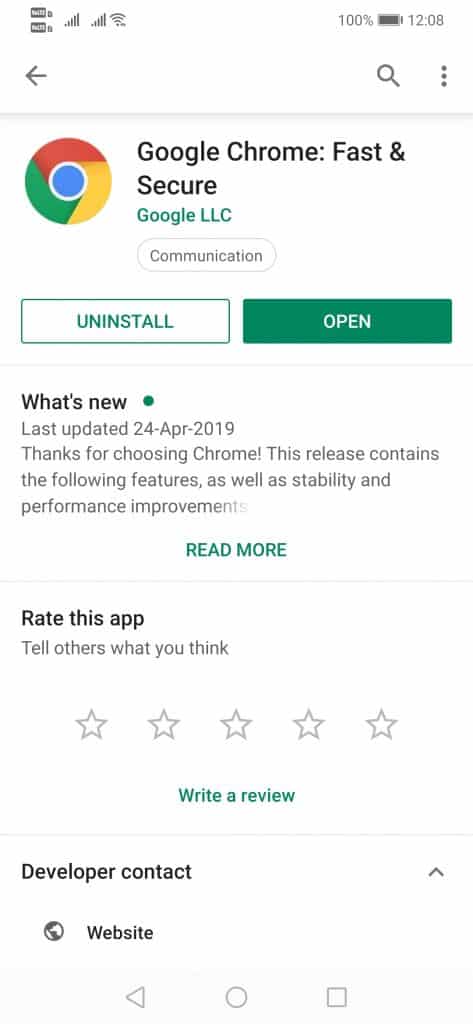The image is a mobile screenshot captured at 12:08 PM, with the device fully charged at 100% and connected to Wi-Fi, indicated by several bars on the Wi-Fi icon on the left. The screenshot displays the Google Chrome app installation page. At the top, the app name is visible: "Google Chrome: Fast & Secure" with the developer, "Google LLC," listed in green beneath it. The Google Chrome icon, a circle with segments colored red, yellow, and green surrounding a smaller blue circle with a white border, is prominently displayed.

Two buttons are visible: a gray "Uninstall" button and a green "Open" button. Below these, there is a section titled "What's New," marked by a green dot, indicating recent updates. The text reveals that the last update was on April 24, 2019, and thanks users for choosing Chrome, mentioning that the release includes new features along with stability and performance improvements, with a "Read More" link in green for additional details.

Further down, the page prompts users to rate the app, encouraging them to "Tell others what you think," accompanied by five gray stars and an option to "Write a review." Under the user review section, there is a "Developer Contact" area featuring the word "Website" next to a gray Earth logo.

At the very bottom of the screenshot, the navigation bar displays three familiar shapes: a triangle, a circle, and a square, representing the back, home, and recent apps buttons respectively.